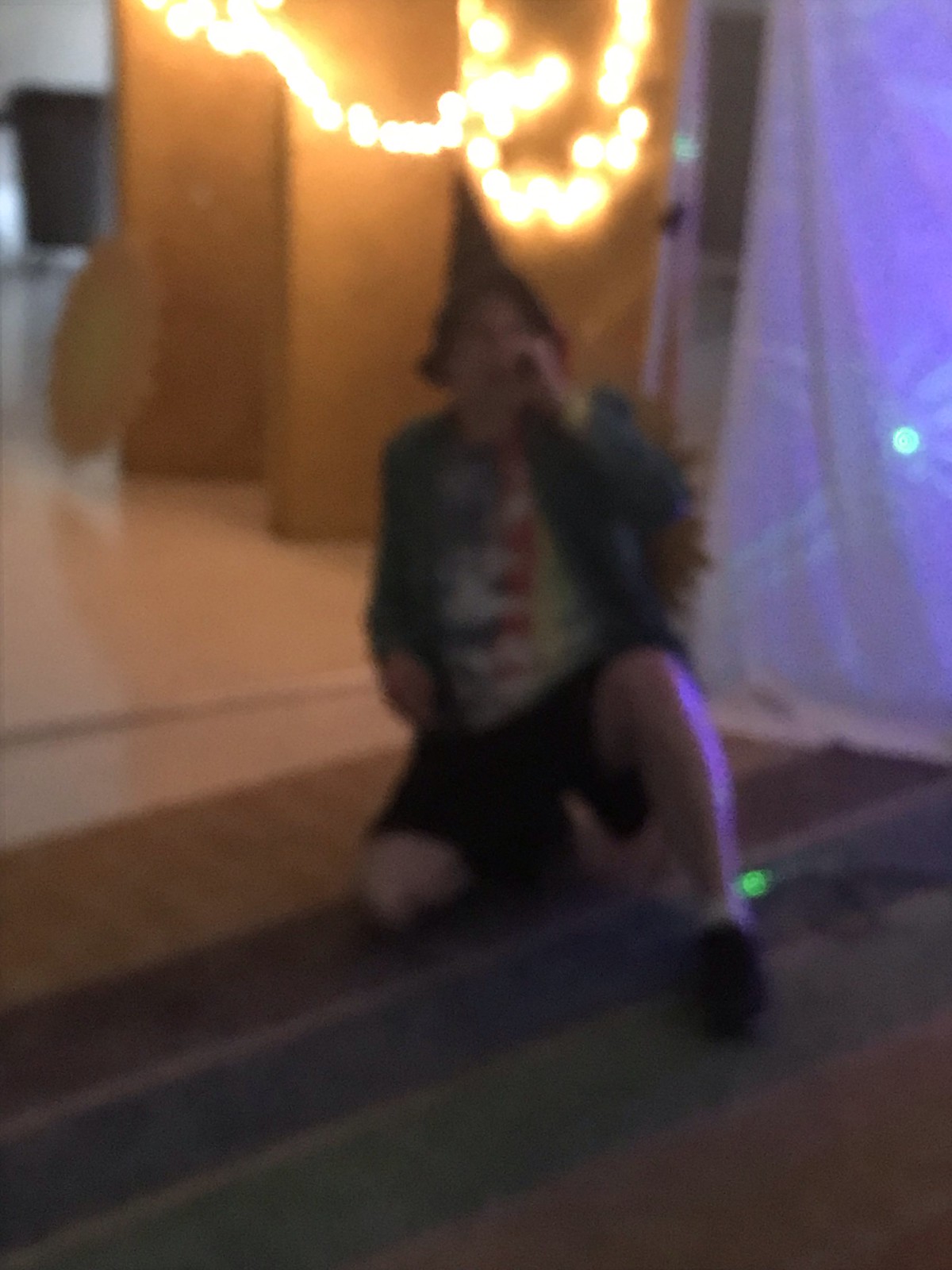In this grainy and somewhat blurry photograph, a light-skinned individual is depicted kneeling on a multicolored rug with shades of gray, blue, green, and orange. The person is dressed in dark-colored shorts, white socks, black shoes, and a grayish top with visible red, yellow, and white graphics. They are also wearing a black or blue long-sleeve shirt and a pointed black hat that resembles a witch's hat. The individual appears to be holding a black microphone, suggesting they might be performing or singing. Behind them, there is a light wood floor section partly visible beneath their knee. The background includes illuminated white string lights hanging above, casting a warm glow. Additionally, there is a yellowish-brown wall or screen, a violet or blue curtain on the right, and some sections that resemble white floor steps. The person's shadow is cast on the flooring, and by their elbow, a green light reflects off a hung sheet onto the floor.